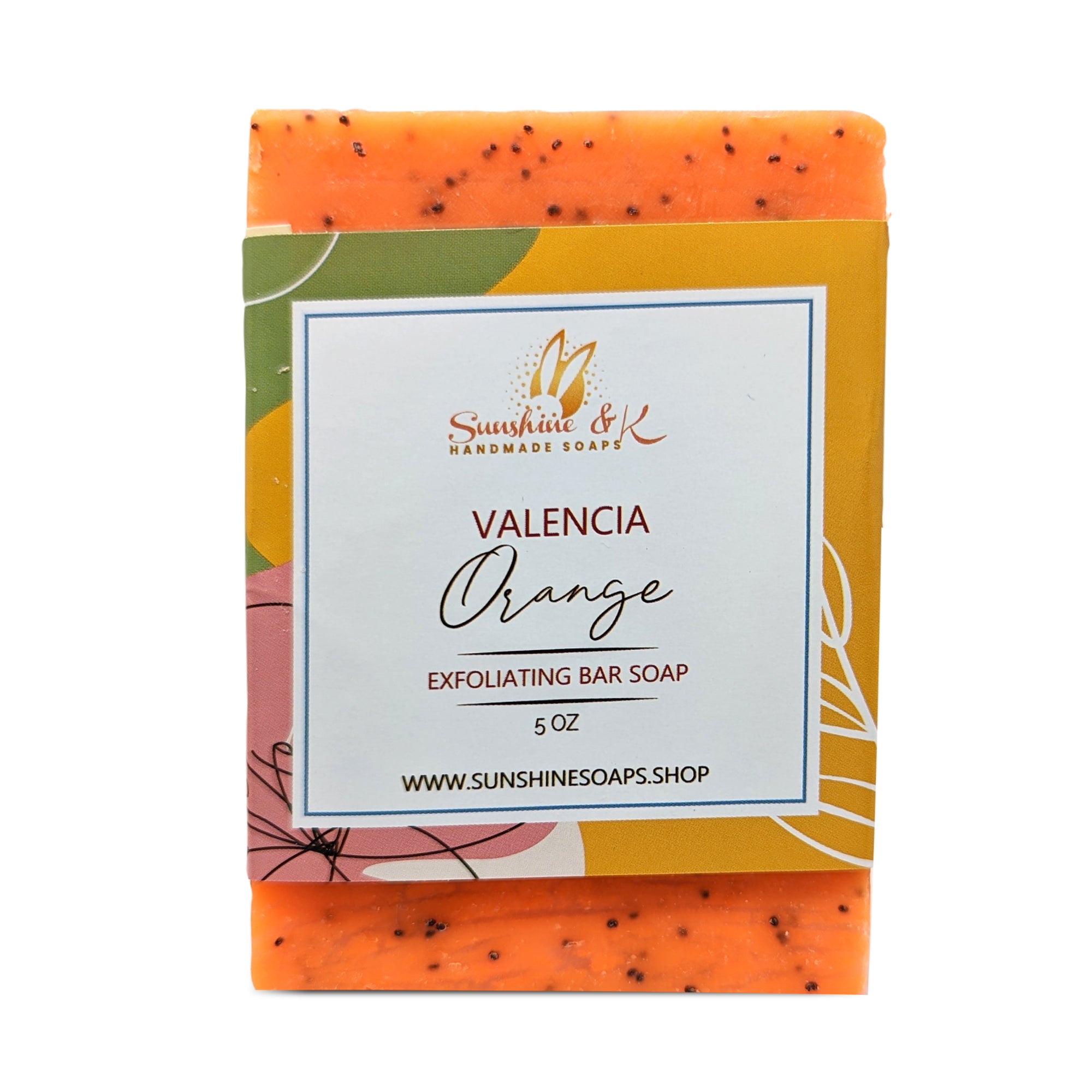This detailed color photograph, in portrait orientation, features a handmade cleansing soap titled "Sunshine and K." The bar itself is a vibrant orange speckled with what appear to be poppy seeds, indicating its exfoliating properties. A wide paper label wraps around the middle of the soap bar, prominently displaying branding and product information. 

The label's design is particularly striking, with a white center panel bordered by abstract, multicolored swirls—dark green at the top left, gold on the right, and pink at the bottom left. At the top of the white panel, "Sunshine and K, Handmade Soaps" is printed, accompanied by a charming logo featuring bunny ears above the word "Sunshine." Below this, the label reads "Valencia Orange" in a mix of standard and script fonts, followed by "Exfoliating Bar Soap" in the center. The weight of the soap, "5 OZ," is listed next, and the URL for the maker, www.sunshinesoaps.shop, is at the bottom in black text.

The photograph showcases the soap in a realistic, representational style, emphasizing the artisanal quality and detailed labeling of this 5-ounce exfoliating bar soap.